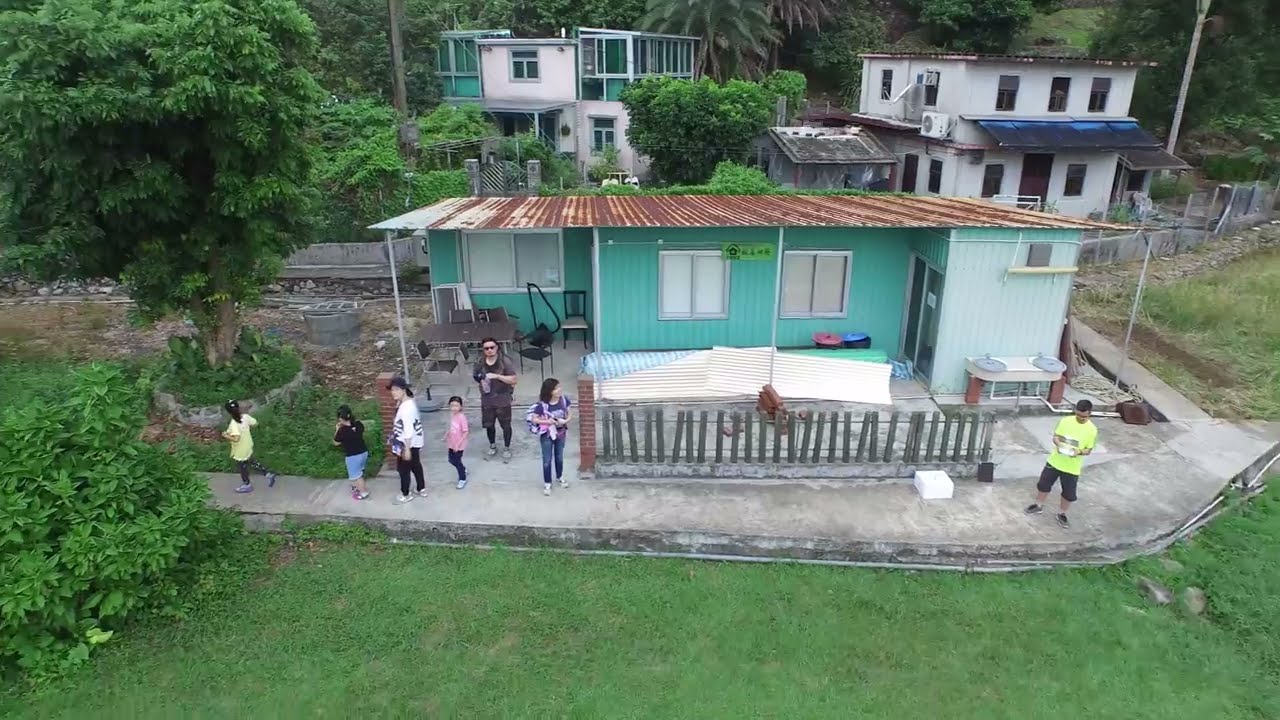In the image, an aerial view captures a quaint, vibrant neighborhood scene. Six people, comprised of three adults and three children, stroll along a concrete sidewalk that meanders through the area. The adults, dressed in black and white shirts, lead three children wearing shirts in yellow, pink, and blue. The group is positioned towards the left of the path, framed by lush greenery with trees and shrubs.

In the foreground is a well-maintained lawn with bright green grass. Dominating the backdrop, there are three distinct homes. The closest home, to the right of the people, has a turquoise-colored exterior with a rusted tin roof, lending it a somewhat rustic charm. Further back, a bi-level white house stands, contrasting with its surroundings. Beyond that, another tri-level house is partly hidden among the trees, exhibiting a mix of white and turquoise with multiple glass-paneled sections reminiscent of greenhouses.

The entire scene unfolds in daylight, under a bright sky, adding a cheerful ambiance to this charming little neighborhood, as if captured by a drone from above.